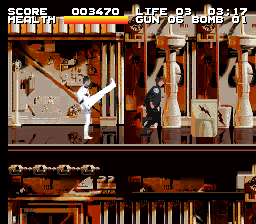This image is a still frame from the older Nintendo video game "Timecop." The screenshot displays a heated moment within a decaying urban environment characterized by a series of columns and deteriorating buildings in the backdrop. 

In the foreground, there are two distinct horizontal levels, the upper one featuring a shiny, brownish floor that reflects the surroundings. On this level, a man in a white karate uniform with a black belt is captured mid-action, performing a high kick with his right leg extended while his left leg remains grounded. The target of his kick is a figure in a black police uniform who appears to be running away.

Additional game interface details are visible at the top of the screen, including the score of 3470, a life count of 3, a time reading of 3 minutes and 17 seconds, a full health bar, a gun count of 5, and a bomb count of 1. The image also features gold and white stripes across the top, enhancing the retro aesthetic typical of the time period.